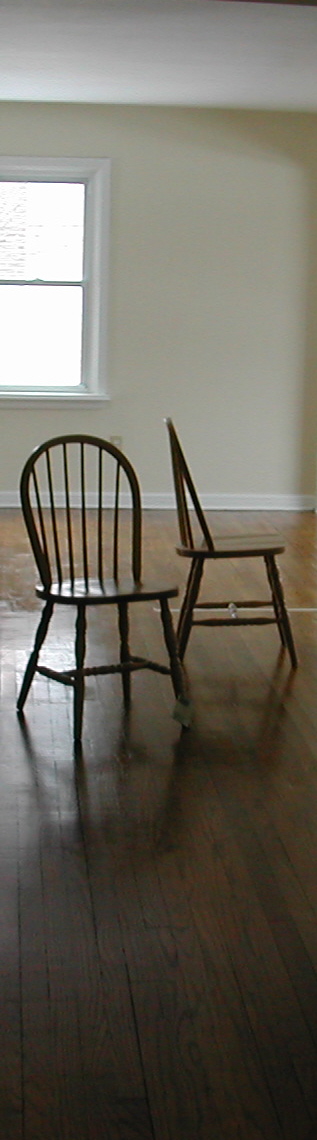This vertically-oriented photograph, resembling a long, narrow slice, captures an indoor scene showcasing a mostly empty room. The room features honey-colored hardwood floors, transitioning to darker brown towards the foreground. The cream-colored walls complement the white ceiling and white floor molding. Centrally placed within the image are two wooden dining chairs with round backs and vertical slats, evocative of farmhouse-style chairs. One chair sits to the left, angled slightly toward the bottom right corner and closer to the camera. The other chair is positioned further back on the right, turned to the right. A window with white trimming, partially cut off by the camera view, allows bright sunlight to filter in, casting shadows of the chairs onto the floor. Beneath this window, there is a barely visible outlet on the wall, and a subtle white line extends across half of the floor behind the right-turned chair.